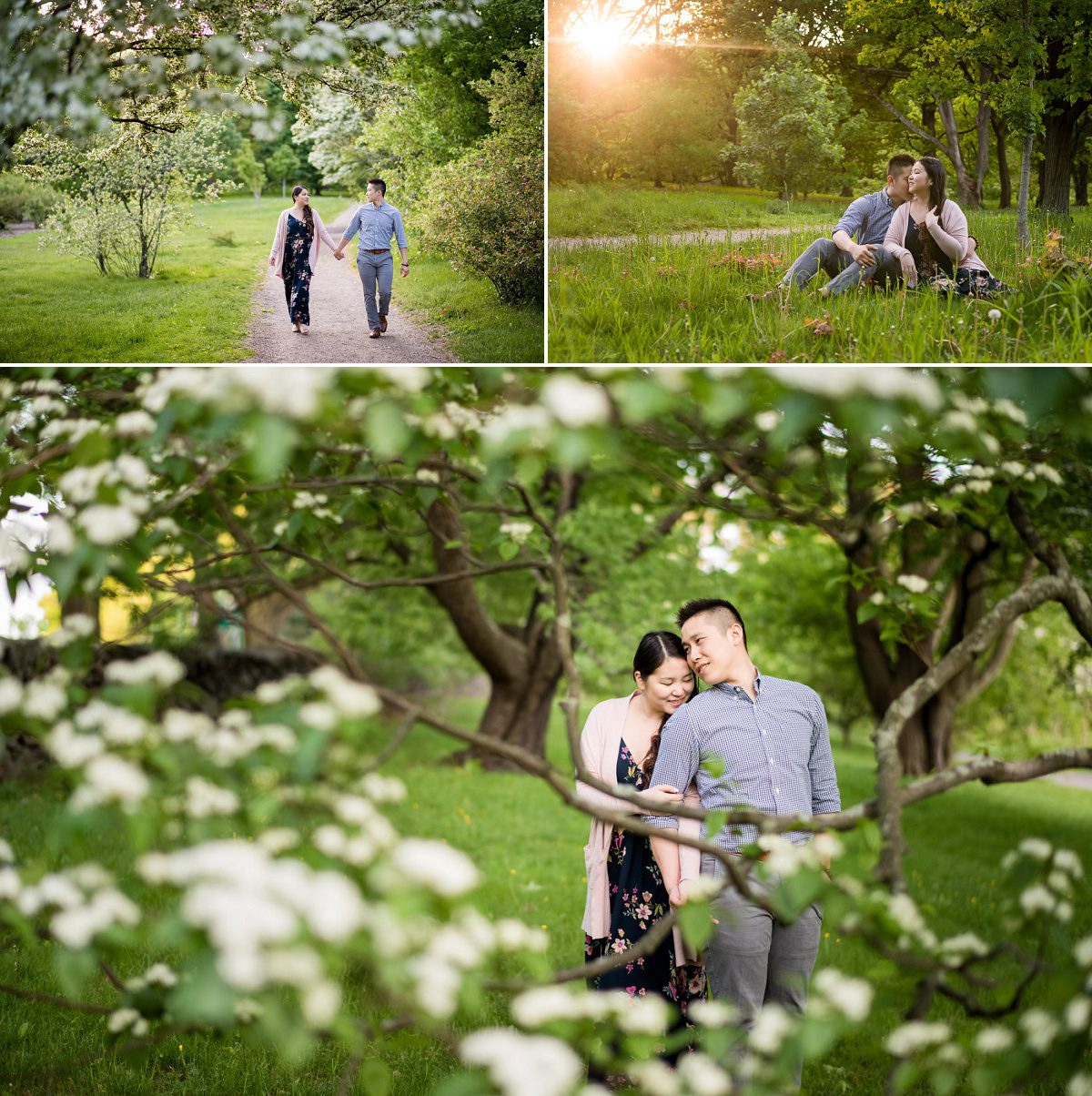This is a professionally taken color photo collage featuring an intimate couple's outdoor photo shoot, likely meant as engagement photos. The collage consists of three photos, with two smaller images on the top and one larger image on the bottom. All the photos capture the couple amidst a serene park setting in the afternoon, bathed in soft sunlight.

In the top left photo, the couple is walking down a gray path lined with lush grass and trees, holding hands and gazing lovingly at each other. The woman wears a dark bluish-green long dress with a floral design, and the man is dressed in a long-sleeve blue shirt and jeans.

In the top right photo, the couple is seated in a grassy field with green trees in the background, giving off a leisurely, affectionate vibe.

The bottom photo, which is the largest, finds the couple standing close to one another, surrounded by trees with delicate white blossoms. The woman is dressed in a black V-neck dress with pink flowers and green leaves, complemented by a long, open cream-colored cardigan, while the man opts for a gray button-up shirt and darker gray pants. They embrace tenderly, encapsulating the romantic and loving atmosphere of the shoot.